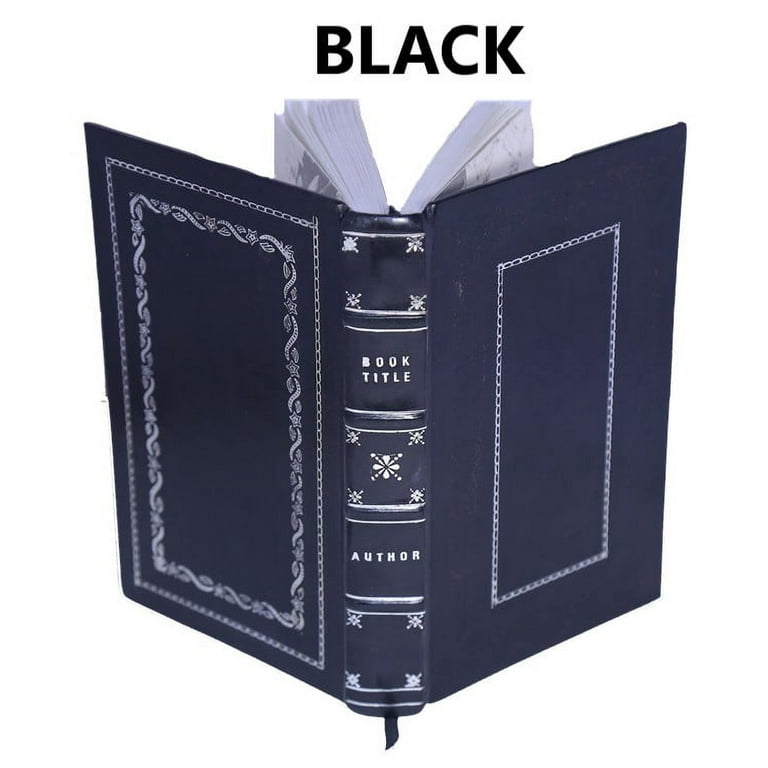This image features an open navy blue book with a blue bookmark string hanging from its bottom edge. The book's spine, visible in the photo, is segmented into five parts, separated by pairs of white lines. The first and third sections feature delicate floral decorations in the corners, with a prominent flower symbol at the center of the third segment. The second section displays the placeholder text "Book Title" in white letters, while the fourth section reads "Author." The front and back covers also have intricate, swirly line patterns forming squares as part of their design. The open book's pages are divided into two main chunks, fanning outward from the center. The entire setup appears to be on a white background, adding contrast to the navy blue book.